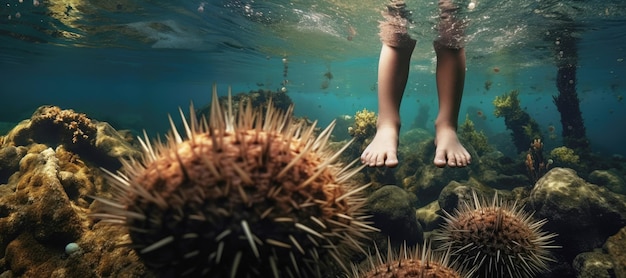This is a detailed underwater photograph, possibly AI-generated, showcasing a serene underwater scene. The focus is on a pair of human feet, submerged up to the knees, with the knees remaining above the water's calm surface. These feet are hovering just above a bed of gray and brown rocks that spread throughout the image. Around these rocks are peculiar, sizeable spiked balls resembling oversized sea urchins or abstract, virus-like shapes. Among the rocks, there are also green, coral-like plants adding to the underwater flora. The water appears to be blue and clear, with minimal disturbance, featuring bubbles and faint ripples. The overall image holds a tranquil composition, with an elongated, horizontal aspect ratio of 1 to 2.